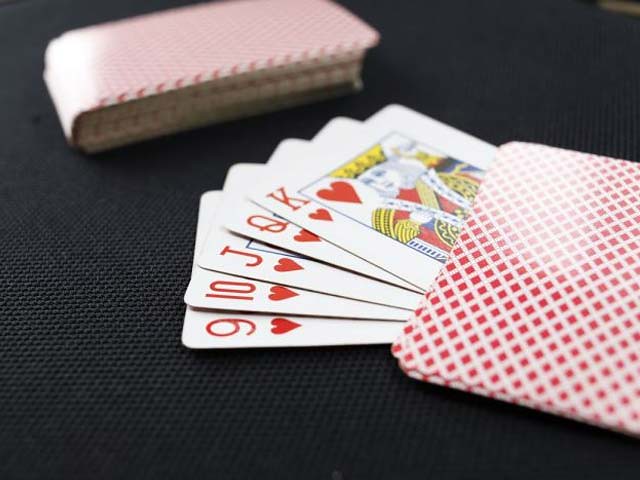In this photograph, a collection of playing cards is carefully arranged on a slightly rectangular, black surface that appears to be made of a grainy or fabric-like material, possibly cloth or carpet, with a subtle pattern of tiny holes. The cards themselves have a slick and glossy finish, adorned with a red and white pattern of intersecting diagonal lines that create a diamond-shaped design, giving the back of each card a distinctive checkered appearance.

On the right side of the image, there is a sizable stack of face-down cards. The top card of this stack catches a hint of light on its left corner, adding a glint to the scene. Beneath this stack lies a perfectly arranged royal flush—five face-up cards from left to right are the nine of hearts, ten of hearts, jack of hearts, queen of hearts, and king of hearts, showcasing a powerful and rare hand in poker.

Towards the upper left corner, there is another neatly stacked pile of face-down cards, positioned in a way that no individual cards are visible. Light also reflects subtly on the left half of this pile. The arrangement leaves a clear space in the upper right and lower left corners of the image, emphasizing the central focus on the cards and the surface upon which they rest.

This meticulously detailed photograph captures the elegance and strategic intrigue of a classic card game, with every element in place to draw the viewer's eye to the intricate design and arrangement of the playing cards.